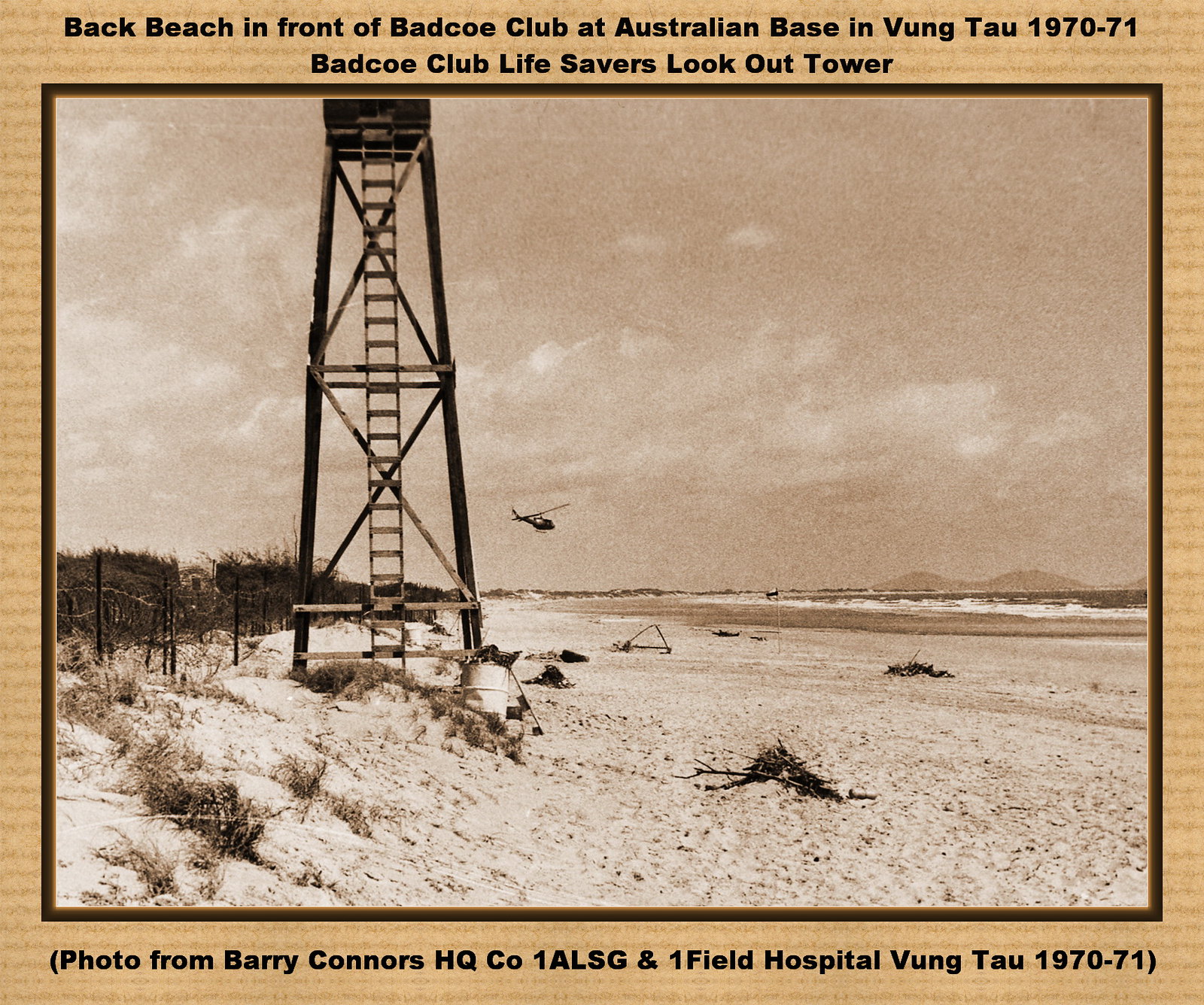This black-and-white photograph, accented with a cream-colored border, captures an evocative scene from the Vietnam War era, specifically between 1970 and 1971. The focal point is the Back Beach, located in front of the BADCO Lifesavers Club at the Australian base in Vung Tau. Dominating the left side of the image is a watchtower equipped with a long ladder, identified as the BADCO Lifesavers Club Lookout Tower. A U1-H1 helicopter is visible flying in the background, emphasizing the military context. The sandy beach extends to the right, merging with the ocean where high waves are visible. In the far distance, across the water, higher hills and peaks rise against the horizon. Vegetation can be seen to the left of the tower, adding a natural element to the landscape. The photograph, sourced from Barry Connors of HQ, 1ALSG, and Ornefield Hospital, captures a poignant slice of life during the war, highlighting both the serene and tumultuous aspects of this historical period.